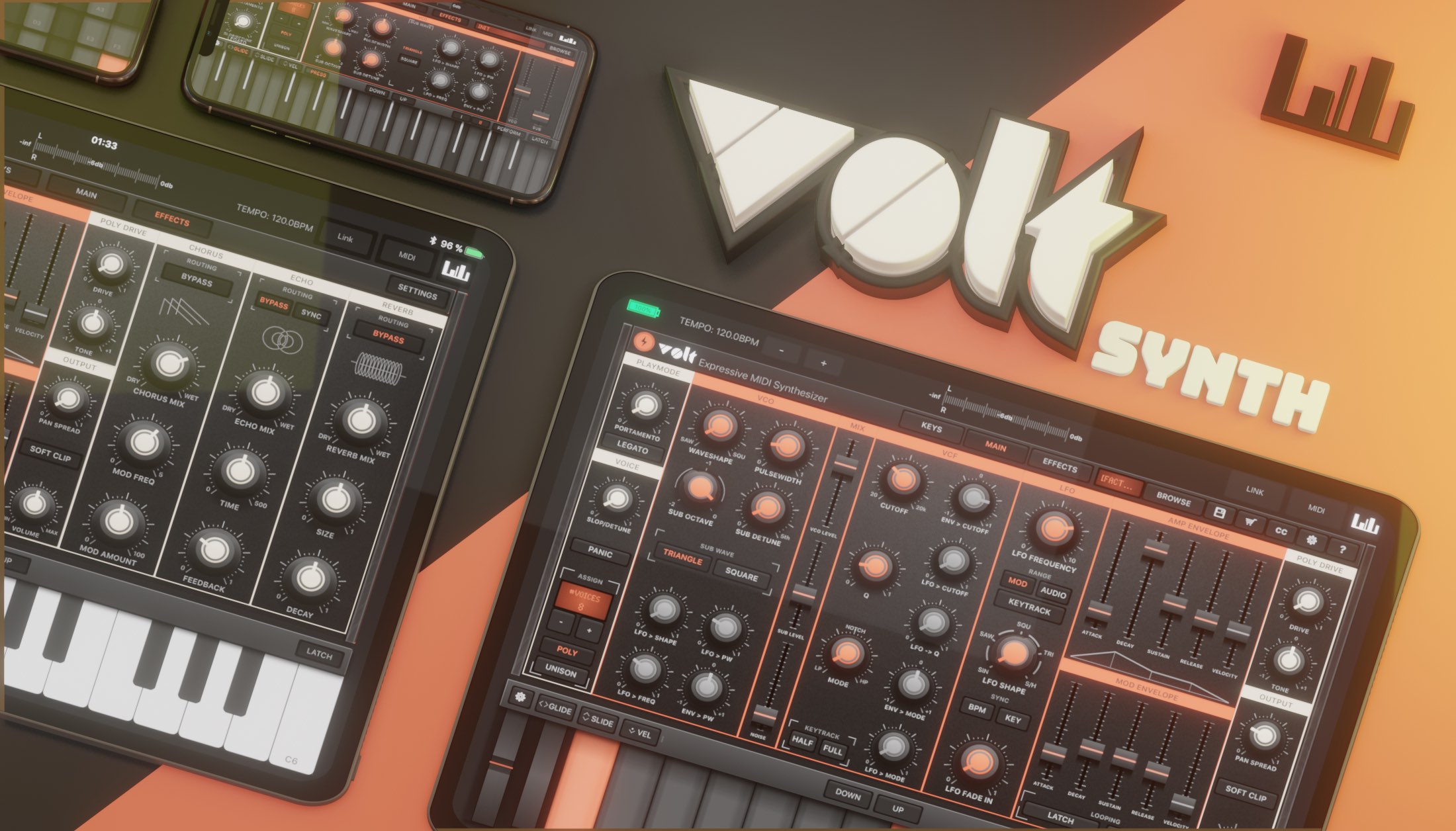A detailed setup featuring various DJ or event equipment is depicted. In the top left corner, multiple horizontal bars with spaces between them are arranged. The sequence includes long, short, long, tall, and short bars, slightly slanted to the right. Central to the setup is the word "VOLT," stylized with an upside-down triangle for the "V" and filled-in "O," all in white with a black outline. To the right, in smaller all-capital letters, it reads "SYNTH."

Below this, two tablets or phones are positioned side by side. The top right section features two horizontal devices. The tablet on the right showcases numerous buttons, resembling a DJ or sound production interface. The tablet on the left displays a keyboard and various switches. Above these devices, the phone on the right mirrors the DJ interface setup, while the phone on the left shows a grid of gray squares.